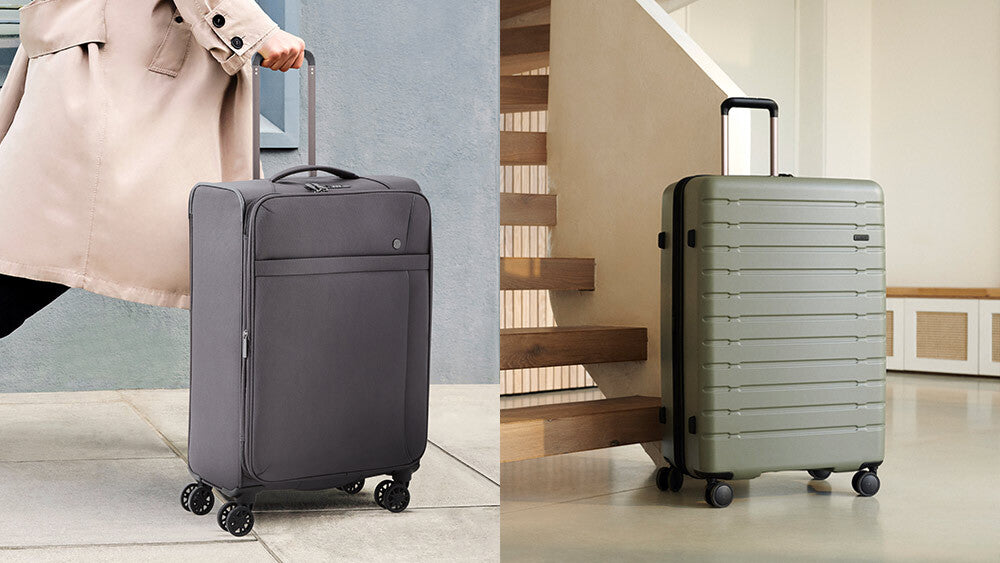The image is a rectangular, horizontal picture divided into two panels, each depicting a separate piece of luggage on a white tile floor. On the left panel, a person wearing a light tan coat is pulling a gray fabric suitcase with compartments, a black top handle, and wheels. The suitcase handle is extended and held in the person's right hand. The left side of the image also features a partial gray wall and some wooden steps leading upwards, indicating that the scene is inside a house.

The right panel showcases a green composite luggage bag with wheels and an extended handle. The bag is standing alone on the white tile floor, positioned near the white wall with a white border and more wooden steps visible to the left. Both suitcases are similarly structured, with functional handles and mobility features, but differ in material and color.